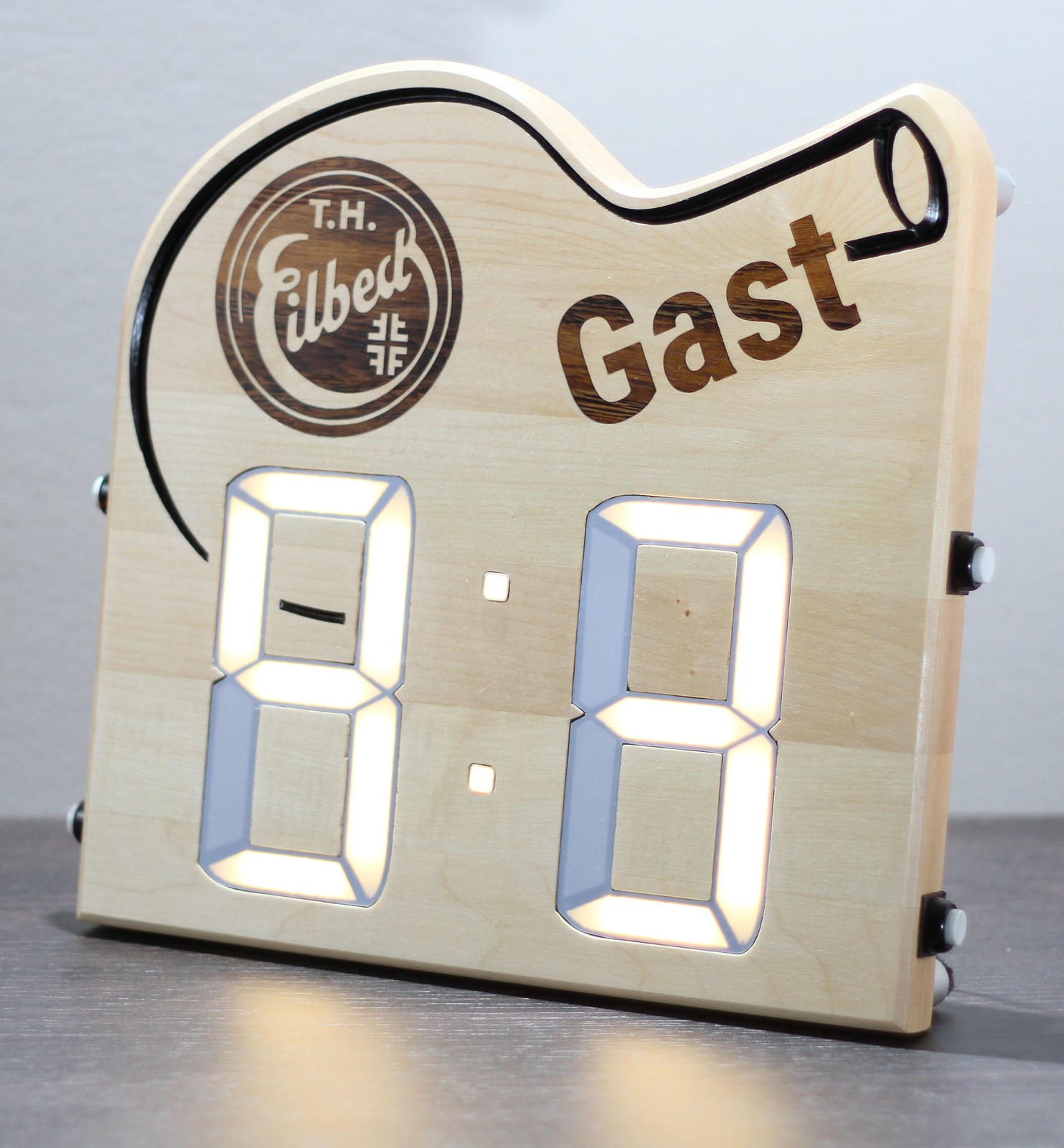The photograph captures an intriguing wooden device placed on a dark gray surface against a light gray wall. The object, predominantly square with a rounded top, features a stylized bottle shape burned into the light blonde wood. A notable black pinstripe outlines the bottle, focusing attention on its unique design. The device prominently displays the text "THEILBECK" and "GAST" in dark brown font across its surface. At the bottom, large white backlit numbers "9.3" are visible, suggesting the device might function as a clock. Each side of the device features small black and white electrode-like protrusions, totaling four. The context, including shadows and surface details, indicates the photograph was taken indoors.